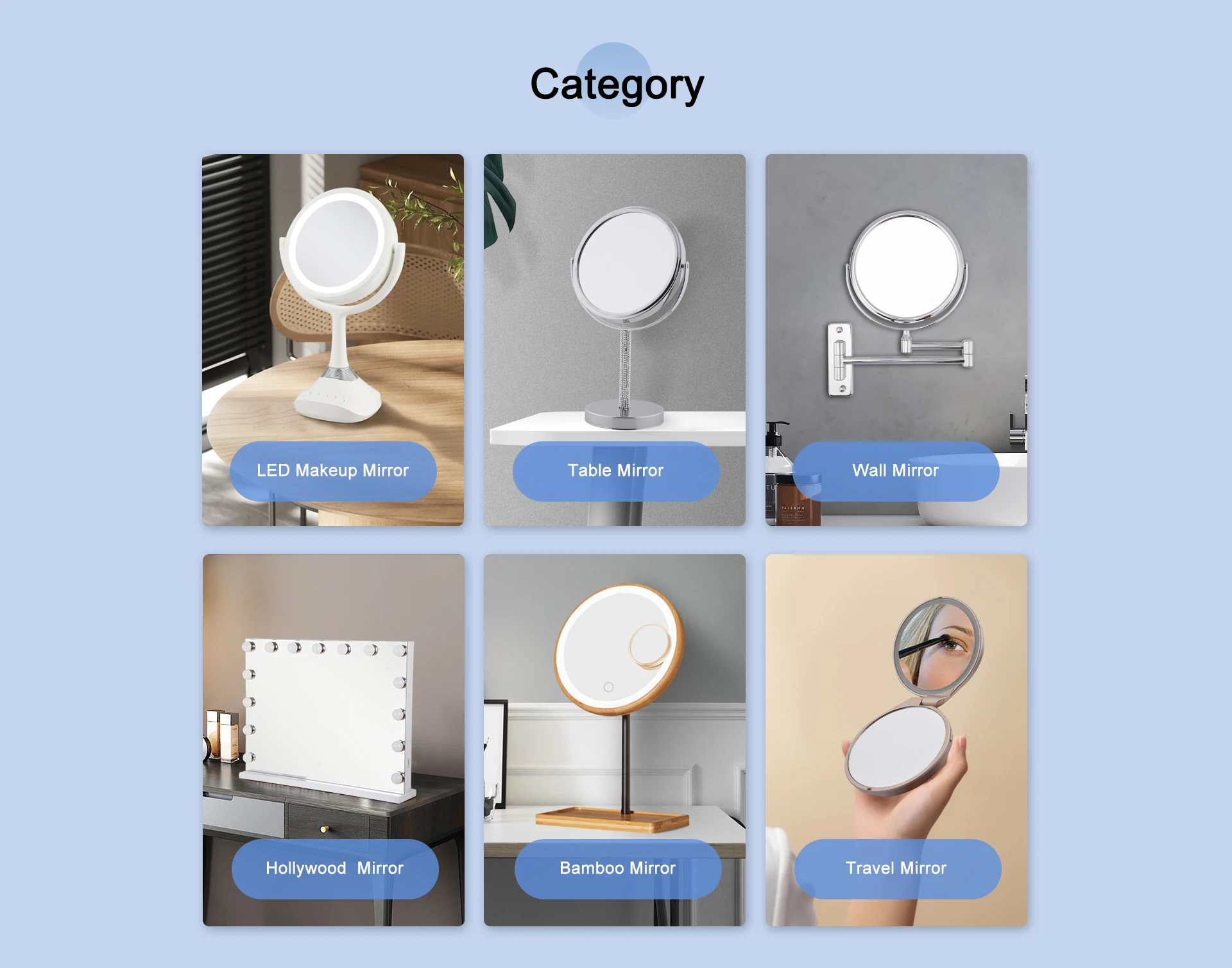The image is a screenshot of product categories from a website. The background presents a subtle gradient, transitioning from purple to light blue, centered. Dominating the composition is a circle with the word "Category" elegantly inscribed in black text.

Arranged in a neat two-row, three-column grid, each category is visually depicted with a corresponding image. Starting from the top left, the "LED Makeup Mirror" category showcases a sleek white LED makeup mirror. To its right, the "Table Mirror" category features a classic table mirror. The top right section displays the "Wall Mirror" category, represented by an image of a wall-mounted mirror.

Continuing to the bottom row, the "Hollywood Mirror" category on the bottom left is illustrated by a large square mirror framed with bright Edison bulbs, exuding a glamorous ambiance. Next, the "Bamboo Mirror" category features an eco-friendly design with a mirror encased in bamboo. The bottom right category, "Travel Mirror," is exemplified by an image of a circular travel mirror held in a hand, reflecting a woman's eye and her makeup application.

Each category name is a dark blue, clickable button, providing a user-friendly interface. The background settings of these product images are minimalist and varied: a plain table and chair, a simple wall with a plant, a bathroom sink, and wall paneling, adding contextual relevance to the product displays.